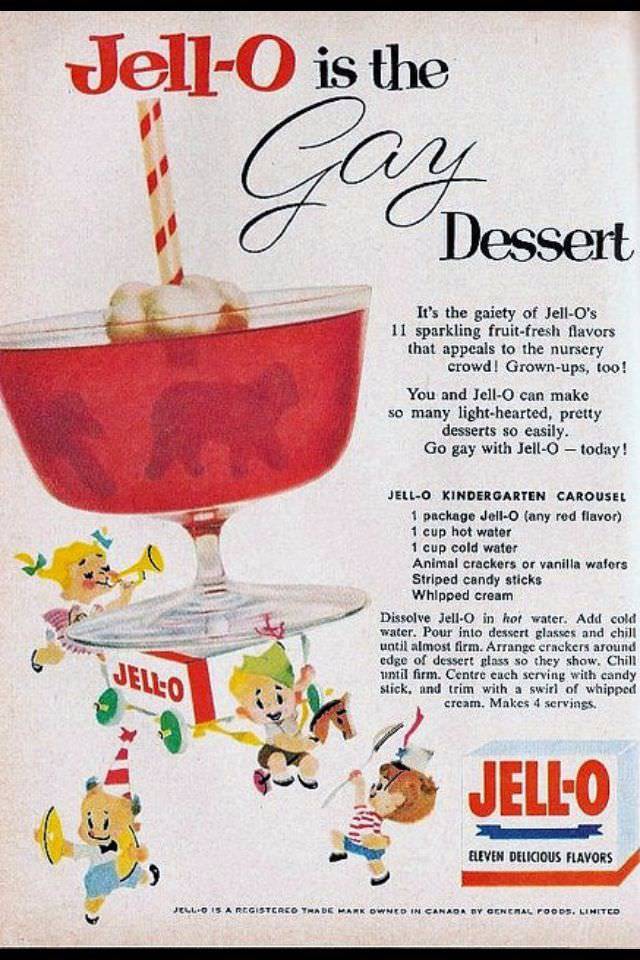This vintage Jell-O advertisement features a playful and colorful design, highlighting Jell-O as "the gay dessert." Centered in the ad is an elegant dish on a stem, resembling a squat wine glass, filled with red Jell-O topped with whipped cream and a candy stick. Surrounding this centerpiece are charming cartoon caricatures of children playing: one rides a rocking horse, another plays a trumpet, a third beats a tambourine, and a fourth marches with a baton. The poster emphasizes Jell-O's appeal to both children and adults with its promise of 11 sparkling, fruit-fresh flavors. Details of a recipe, titled "Jell-O Kindergarten Carousel," are provided, calling for one package of any red-flavored Jell-O, hot and cold water, animal crackers or vanilla wafers, and whipped cream. Instructions explain how to dissolve the Jell-O, chill it until almost firm, arrange the crackers around the dessert glass, and decorate with a candy stick and whipped cream. The ad, framed by black borders on a speckled gray background, sparks nostalgia with its whimsical, old-timey design and cheerful message.